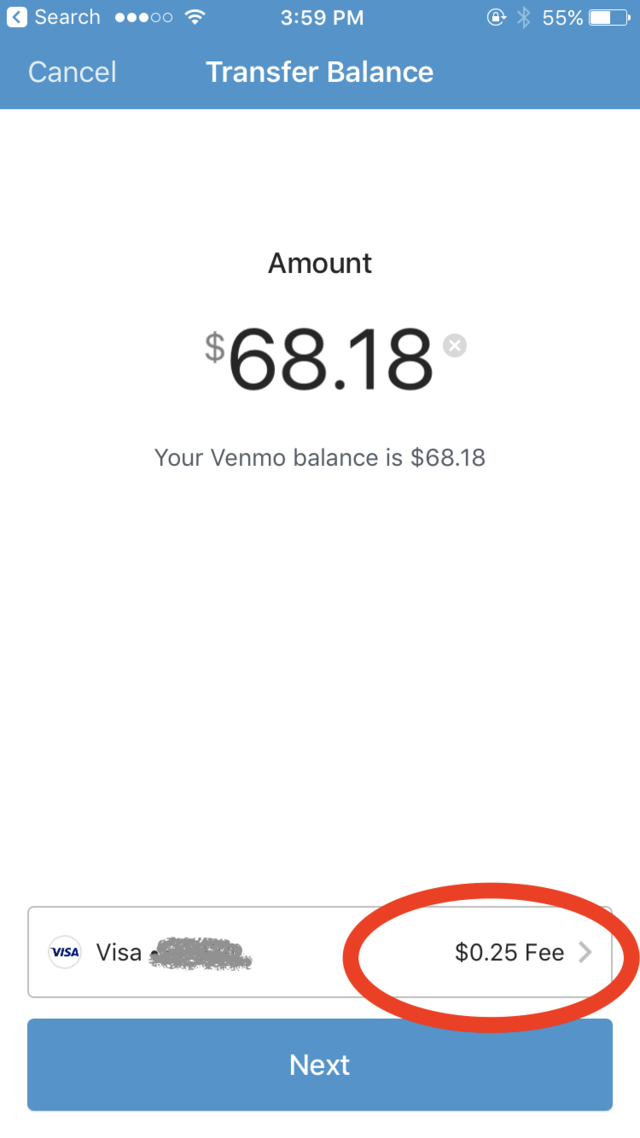This is a detailed screenshot of the Venmo app on a smartphone, captured at 3:59 p.m. At the top of the screen, service indicators are followed by the time in the center and symbols for a lock, Bluetooth, and a battery at 55% on the right. Below this, the header displays "Transfer Balance" prominently in white lettering with a "Cancel" option on the left.

The screenshot reveals that the user is transferring $68.18, which matches their Venmo balance stated just below this amount in smaller black text. At the bottom of the screen, there's a section indicating the transfer destination, which is a Visa card with its number obscured by gray scribbles. Adjacent to this is a note about a $0.25 fee, circled in red, with a small gray arrow to the right.

Below these details, a large blue button labeled "Next" in white text indicates the next step in the transfer process. This image illustrates the user transferring their Venmo balance to their bank account or debit card, highlighting the associated $0.25 fee.